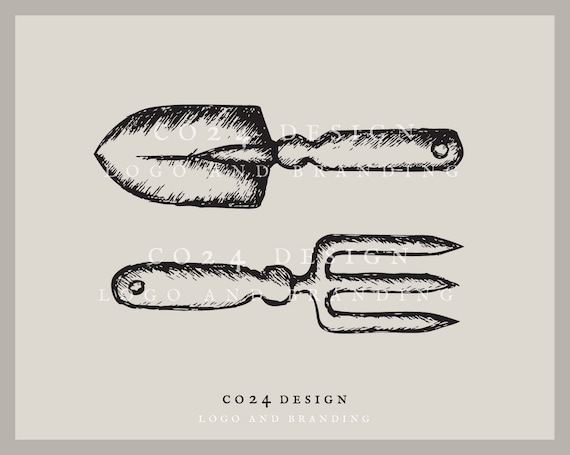This image is a small, horizontal rectangle rendered entirely in shades of gray. There is a dark gray border surrounding a lighter gray background upon which two hand-drawn garden tools are depicted. These tools— a hand shovel and a hand pitchfork with three prongs— are illustrated with meticulous black shading to enhance their details. Both tools have handles designed with small holes at the ends for hanging. Centrally positioned between the tools, the phrase "CO24 design" is written in white, signifying the brand or artist responsible for the image. The same "CO24 design, Logo, and Branding" text, also in white, is repeated at the bottom of the image. The overall aesthetic combines gray tones with a clear focus on branding and design presentation.